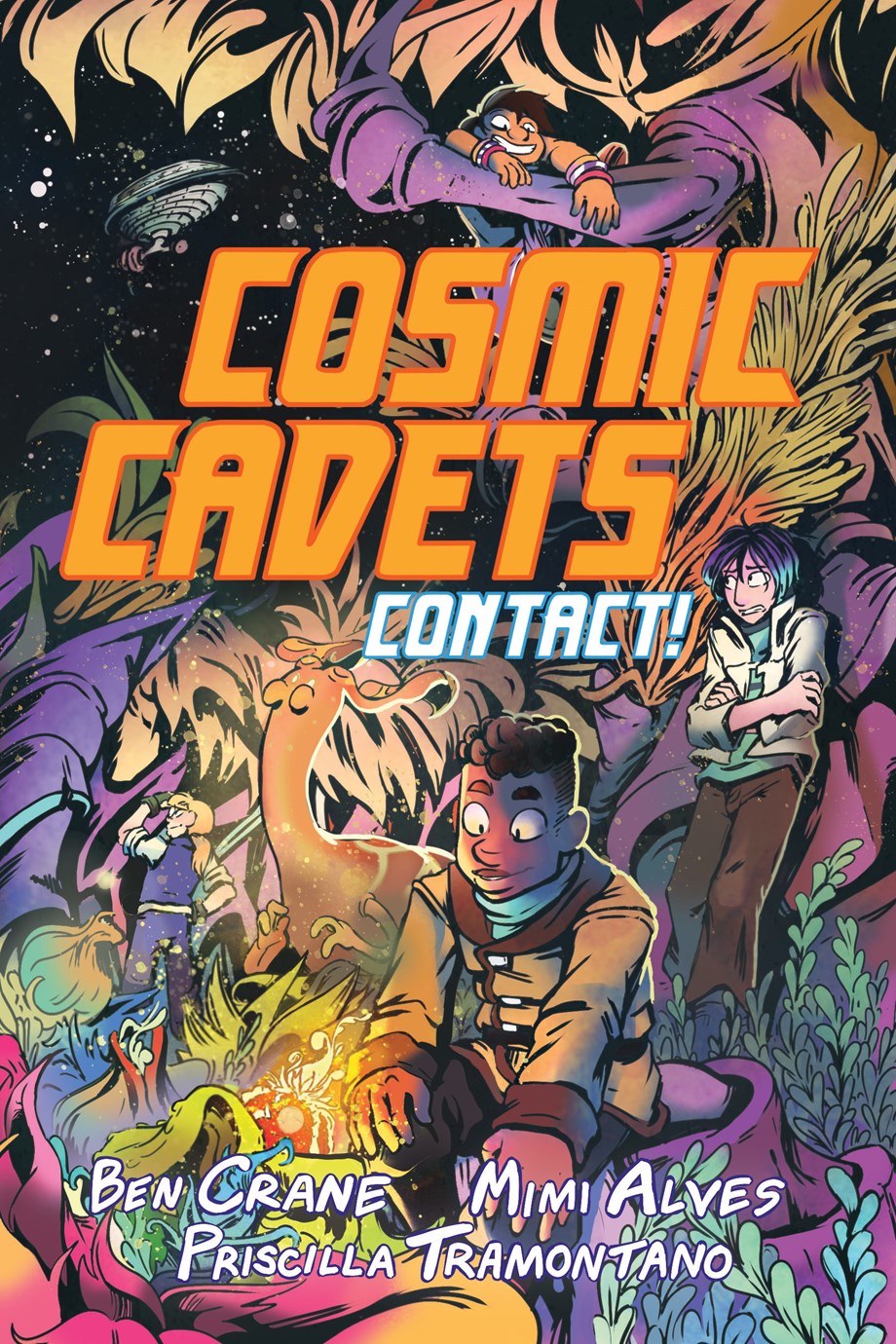The cover of the comic book "Cosmic Cadets: Contact" bursts with vibrant colors and dynamic illustrations, portraying an adventurous scene with four cartoon characters. Central at the bottom, a character with brown skin, curly hair, and a brown jacket sits on a stump, gazing with wonder at a glowing, unusual flower. To the right, another figure, with ambiguous gender, shows a look of fear or cold, arms wrapped around their body, clad in purple and blue hair and brown pants. In the background, a girl with reddish hair, wearing a purple top and matching pants, appears to be looking around for something. To the left, a boy sits near a campfire, large white eyes staring intently. Above, a lively character hangs from a purple tree branch, smiling enthusiastically. The title "Cosmic Cadets" is prominently displayed in large orange block letters, with "Contact!" beneath in white letters with a blue border. The names Ben Crane, Mimi Alves, and Priscilla Tramontano are credited at the bottom, indicating their roles as contributors to this dazzling comic book cover.